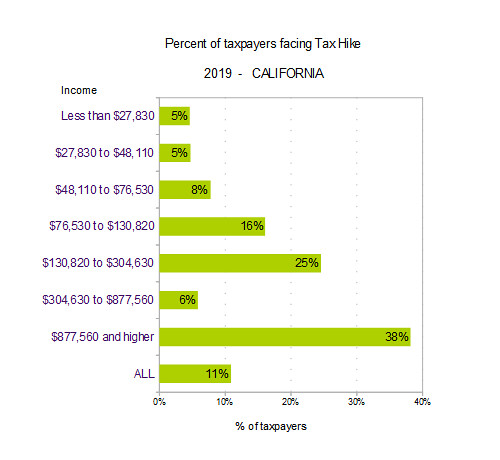The image is a vertically-oriented bar graph titled "Percent of Taxpayers Facing Tax Hike," with a subtitle "2019 - California." The graph features a clean white background encased in a black border. Along the left-hand side, income brackets are listed in purple text: "Less than $27,830," "$27,830 to $48,110," "$48,110 to $76,530," "$76,530 to $130,820," "$130,820 to $304,630," "$304,630 to $877,560," and "877,560 and higher." 

Each income bracket has a corresponding green bar indicating the percentage of taxpayers within that bracket facing a tax hike. Specifically, the percentages shown are: 
- Less than $27,830: 5%
- $27,830 to $48,110: 5%
- $48,110 to $76,530: 8%
- $76,530 to $130,820: 25%
- $130,820 to $304,630: 6%
- $304,630 to $877,560: 38%
- $877,560 and higher: 38%

At the bottom, the overall percentage of taxpayers facing a tax hike in California for 2019 is noted as 11%.